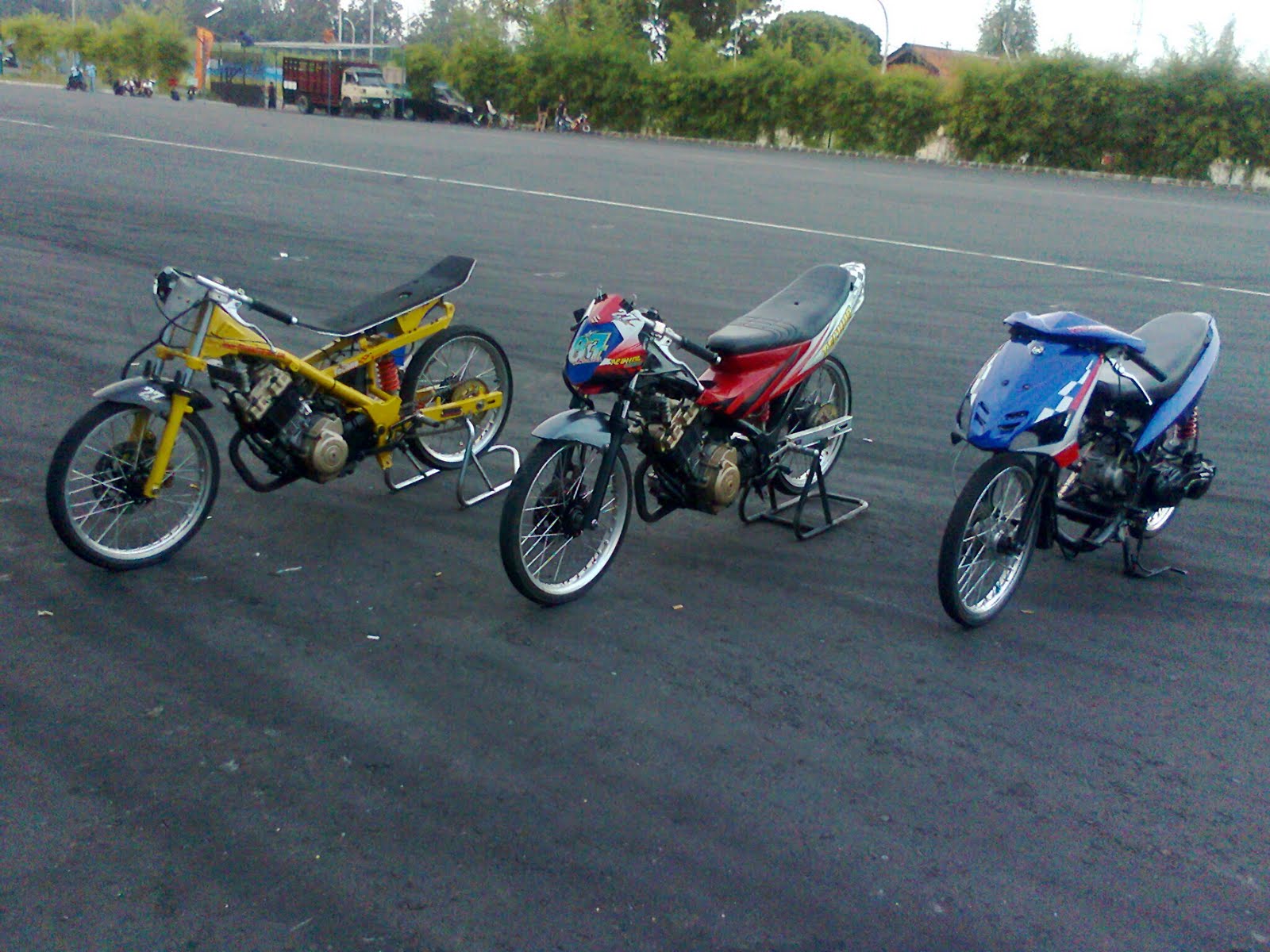The image showcases three off-road motorcycles lying diagonally on a vast stretch of asphalt, occupying the center of the frame. The leftmost bike is yellow and features a flat seat, with the number 22 visible on its wheel. The middle bike sports a red, white, and blue color scheme, while the rightmost bike displays blue, white, and some red accents. The backdrop includes a view of bushes, a beige truck with a red bed, some pedestrians, and the roof of a house, indicating an outdoor setting. This scene could be from a race, a bike show, or simply a candid street photo. The primary colors present in the image are gray, white, black, yellow, red, blue, and orange.